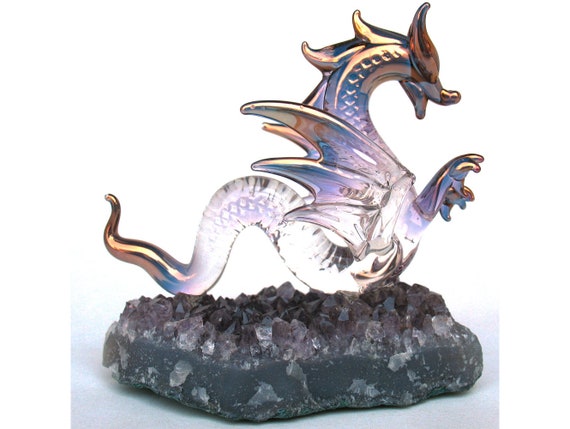The image depicts a detailed, artistic piece featuring a serpentine dragon made of clear, glass-blown material with intricate scale details, perched on a jagged, charcoal gray base with amethyst-colored accents. The dragon's lithe body tapers into a tail, and it possesses two wings that exhibit hints of gold at the tips. Gold tones also accentuate its mouth and mane, adding a striking contrast to the primarily clear structure. The base upon which the dragon rests is comprised of irregularly scattered crystals, with a mix of gray, pinkish, and purple hues giving it an almost cavernous appearance. This carefully crafted artwork combines elements of both fantasy and geology, bringing to life an ethereal scene of a dragon poised on mystical, crystalline rocks against a stark white background.